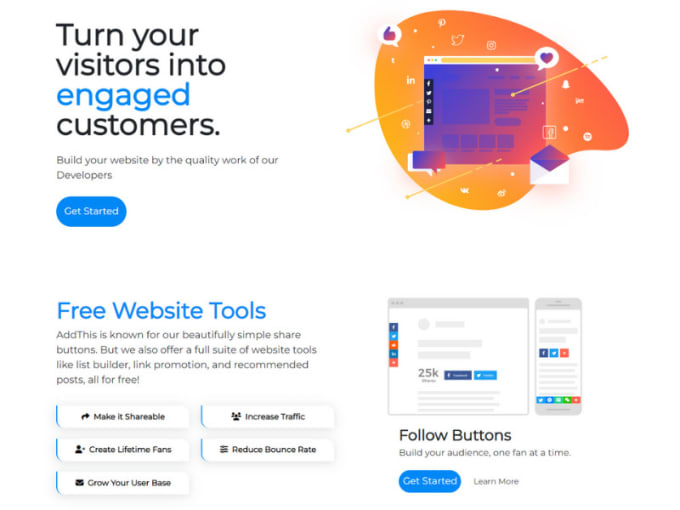The image appears to be a promotional advertisement with a clean and minimalist design. It features a stark white background to emphasize the text and graphical elements prominently. 

On the left side, bold and engaging text reads, "Turn your visitors into engaged customers." Directly beneath this, another line encourages the viewer to "Build your website by the quality work of our developers." These statements are designed to attract potential clients by highlighting the benefits of their services. 

Centered below the text is a prominent blue oval button with white text that says "Get Started," inviting immediate action from the audience.

To the right of the text is an orange graphic in the shape of a paint palette, symbolizing creativity and design. The palette is filled with small white icons including a square representing a webpage, a thumbs-up within a circle, a heart within a circle, a rectangular talk box, and an envelope—alluding to various digital and social media interactions.

Further down, on the left side, the text elaborates on the offerings: "Free website tools." It mentions that "AddThis is known for our beautifully simple share buttons, but we also offer a full suite of website tools like list builder, link promotions, and recommended posts, all for free."

Below this explanation are rectangular boxes containing key benefits: "Make it shareable," "Increase traffic," "Create lifetime fans," "Reduce bounce rate," and "Grow your user base," each one emphasizing different advantages of their tools.

On the right side, there are graphical elements, including a white square with a grey border and a white rectangle with a grey border, each containing various colored boxes, illustrating the diversity and integration of their tools.

At the bottom right, the text promotes "Follow buttons," encouraging users to "Build your audience one fan at a time." Two actionable links, "Get Started" and "Learn More," provide options for further engagement.

Overall, the caption comprehensively describes the advertisement, highlighting its components and the benefits it offers in a succinct, compelling manner.